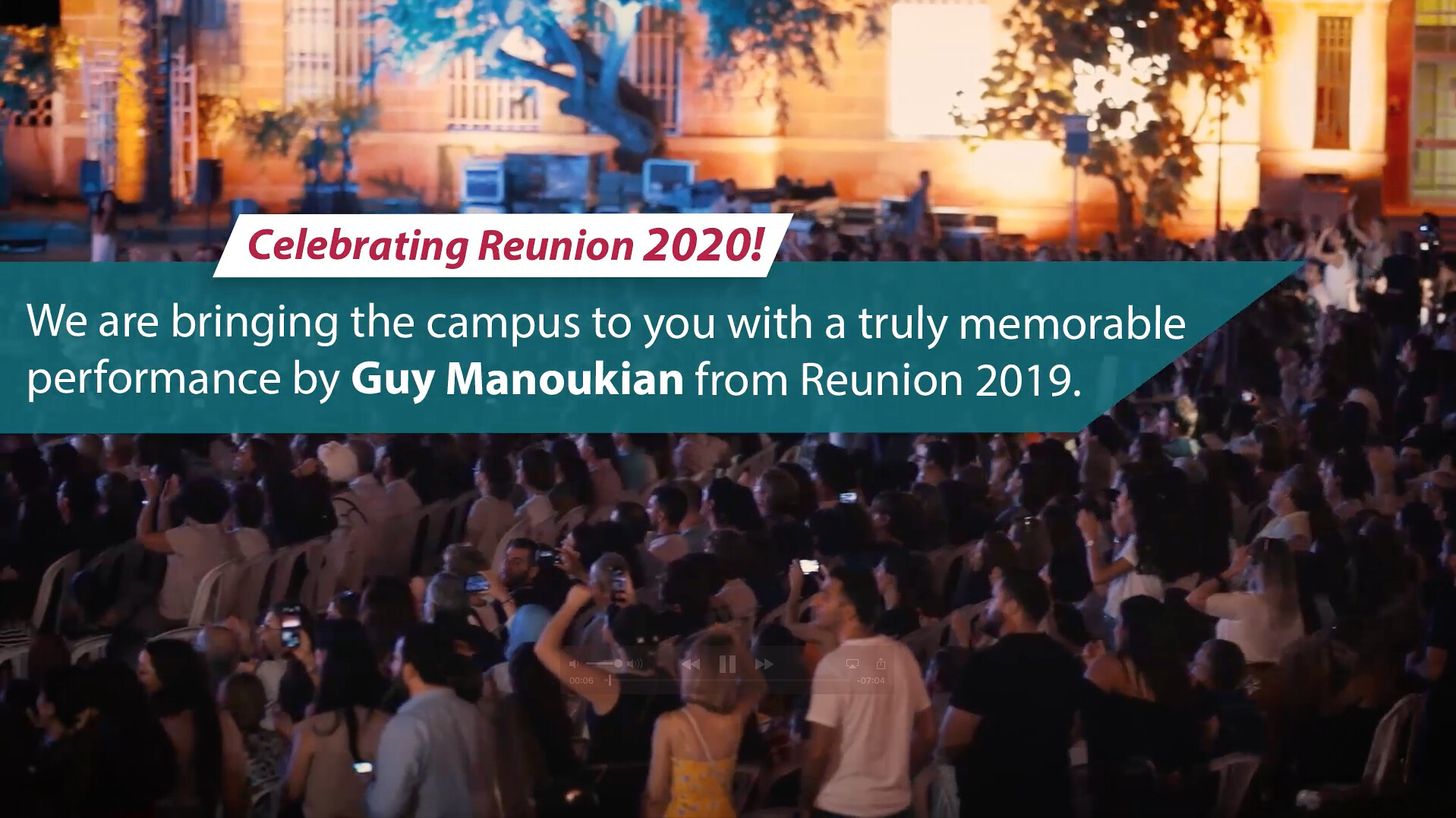The image depicts a large crowd of men and women gathered in front of a substantial, well-lit stone building, possibly for a street festival or a church reunion. The building in the background, illuminated by lights and giving off an orangey hue, features visible windows and doors and is framed by trees. The center of the image is dominated by a blue, semi-transparent banner with white text that reads, "We are bringing the campus to you with a truly memorable performance by Guy Manoukian from Reunion 2019." Above this banner, in red letters against a white background, the text "Celebrating Reunion 2020" is prominently displayed. The audience appears captivated, with many individuals standing or sitting, some taking photos with their phones, enriching the lively and vibrant atmosphere of the reunion event.